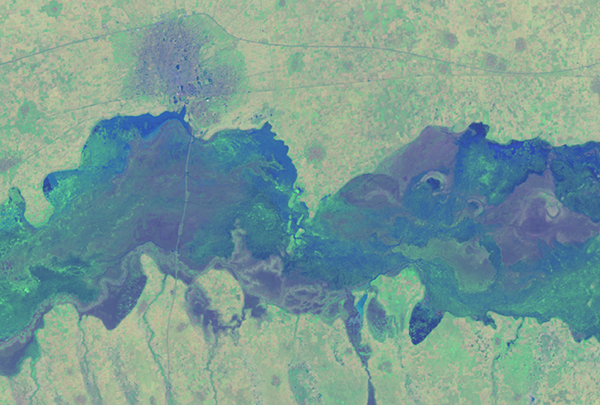The image is an abstract painting primarily dominated by light green and gray hues with dark green and blue accents. At the center, extending from left to right, are striking blue paint splashes, possibly representing a water body, interspersed with light purple and additional light green streaks. The bottom of the painting features predominantly gray areas with occasional light green elements, while the top also showcases a gray background. Two faint light blue lines traverse the painting horizontally. Scattered across the artwork are subtle details, including light gray dots and gray circles, adding depth to the composition. This intriguing piece lacks any text, emphasizing its abstract nature and inviting interpretation, as one might expect to find hanging in an art show.